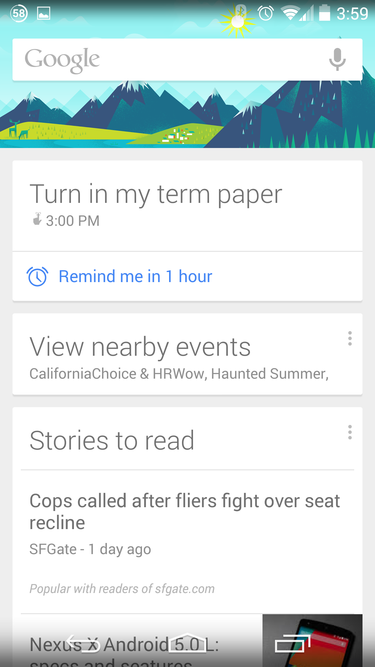A detailed vertical image capture from a Google device interface. In the upper left corner, there's a circular icon with the number "58" inside it. Adjacent to it, on the upper right, is a square icon displaying a cloud image, symbolizing weather. Surrounding these are various status icons: the sun (likely indicating time of day), a clock icon, a Wi-Fi signal symbol, a cellular signal strength indicator, a battery life icon, and the current time displayed as "3:59."

The background of the interface showcases a picturesque scene with snow-capped mountains, green hills, and a sky gradient, typical of a scenic wallpaper. Centered prominently near the top is the Google search bar, featuring the word "Google" in gray text accompanied by a microphone icon on the right.

Below this, a gray box spans the width of the screen with embedded white boxes. The first white box contains a reminder: "Turn in my term paper at 3 p.m." Below it, a separating line leads to a blue clock icon with the text "Remind me in one hour." Following this, another white box suggests local events, listing "California Choice," "HR Wow," and "Haunted Summer."

Further down, another white box titled "Stories to read" appears, featuring a headline: "Cops called after fliers fight over seat recline," sourced from SF Gate one day ago, noted as "Popular with readers of SFgate.com."

At the bottom of the image, partially overlapping icons indicate additional functionalities or tools. The text "Nexus X" and "Android 5.0 L" is visible, though partly cut off. A small phone icon is visible on the lower right side.

This detailed depiction accurately describes a typical smartphone interface with user reminders, news suggestions, and status indicators.